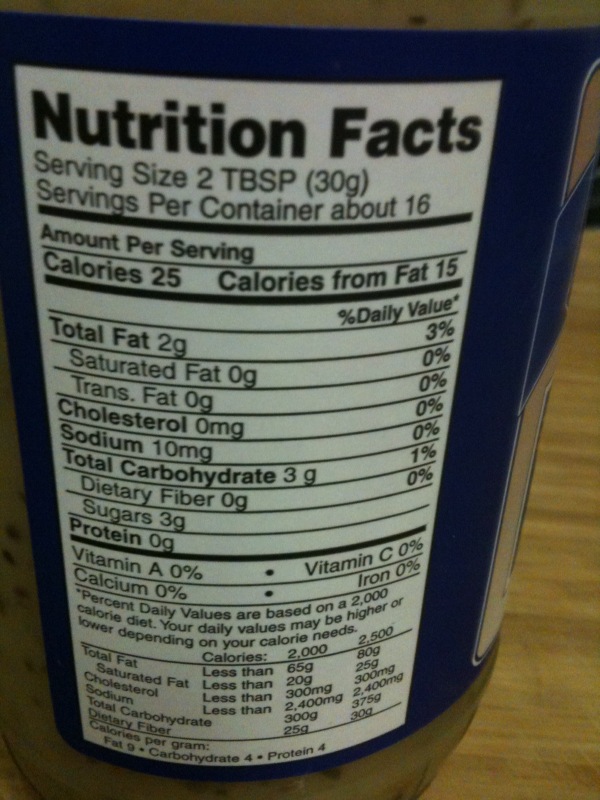This image is a close-up of a nutritional label on a container with a blue border, set against a wooden tabletop background visible on the right and lower portions of the photo. The label, marked "Nutrition Facts," details the serving size as 2 tablespoons (30 grams), with approximately 16 servings per container. It lists the following information: 25 calories per serving, including 15 from fat; 2 grams of total fat (3% Daily Value), 0 grams of saturated and trans fat (0% DV), 0 mg of cholesterol (0% DV), 10 mg of sodium (0% DV), 3 grams of total carbohydrates (1% DV), including 3 grams of sugars, and 0 grams of dietary fiber and protein. The vitamins section shows all zeros: vitamin A, vitamin C, calcium, and iron all at 0%. At the bottom, there's a standard note explaining that the % Daily Values are based on a 2,000-calorie diet and may vary depending on individual calorie needs, with a chart comparing daily values for 2,000 and 2,500 calorie diets. The overall impression of the label suggests that the contents might not be nutritionally robust.